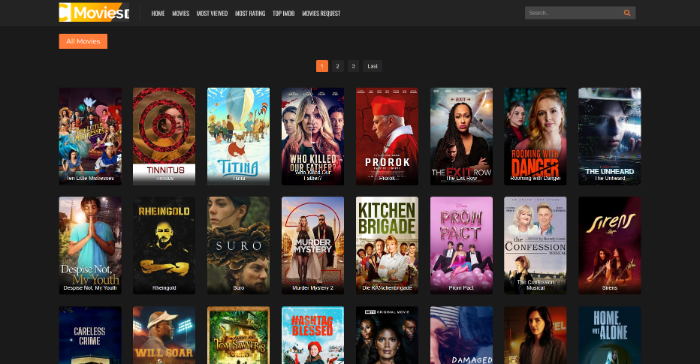This image captures a detailed screenshot of a movie-focused webpage, complete with a navigation bar at the top, featuring clickable options such as Home, Movies, Most Viewed, Most Rated, Top IMDb, and Movie Requests. Below these options is a link labeled "All Movies," followed by pagination links marked as 1, 2, 3, indicating multiple pages of movie content, with page 1 currently active. The movie thumbnails are displayed in a vertical list; the first movie’s title is blurred, but several other titles are visible in order. The second movie is "Tinnitus," followed by "Titina," "Who Killed Our Father," "Pro Roque," "The Exit Row," "Rooming with Danger," "The Unheard," "Despise Not My Youth," "Rango," "Suro," "Murder Mystery 2," "Kitchen Brigade," "Prom Pack," "The Confession Musical," "Sirens," "Careless Crime," "Will Soar," "Tom Sawyers," "Hashtag Blessing," "Damaged," "Home and Alone," and two unnamed movies. Each listed movie presumably leads to additional information and possibly streaming options.